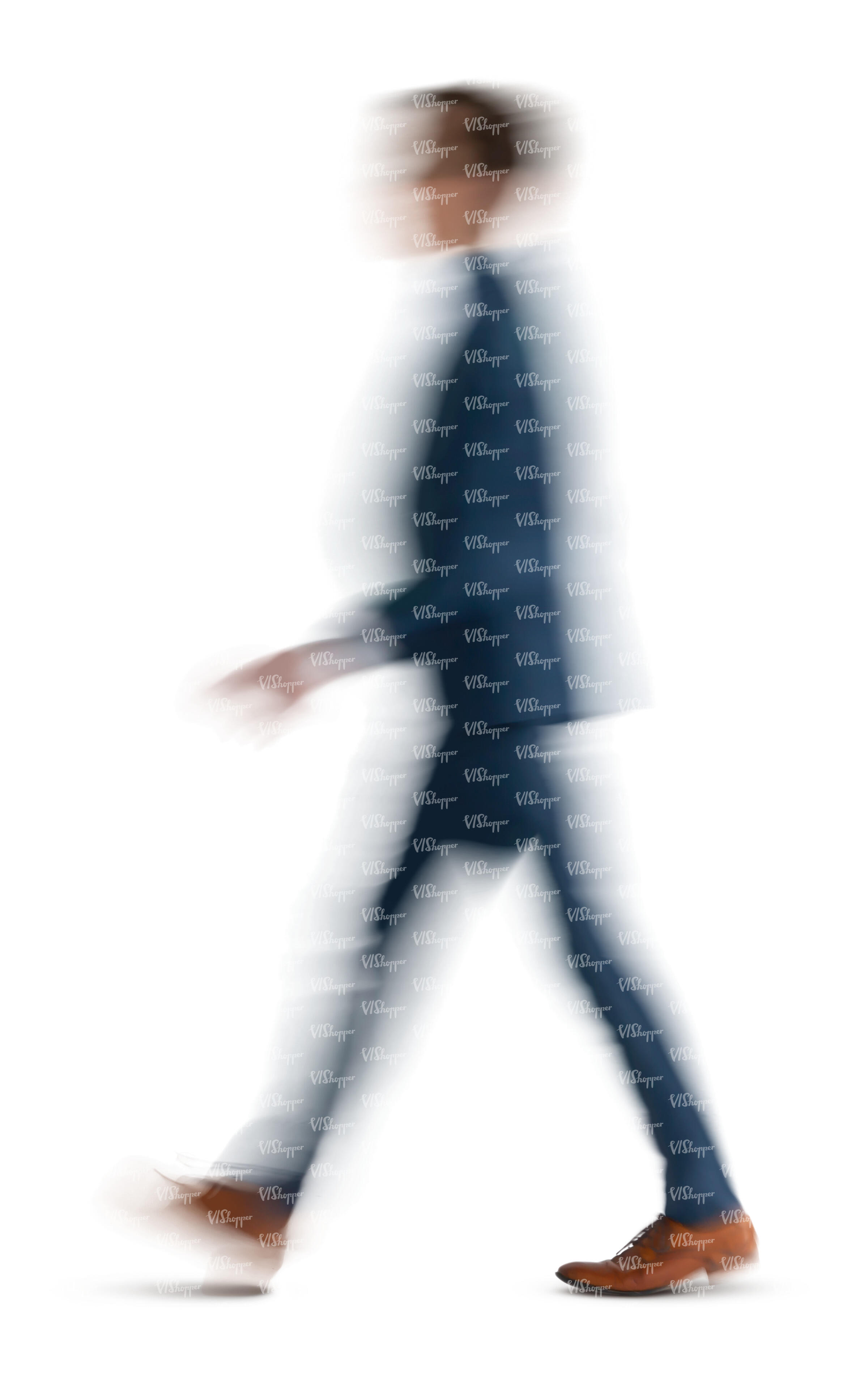The image is a rectangular, intentionally blurred stock photograph depicting a person walking to the left, with their legs spread in motion. The individual is wearing a blue business suit, including a jacket and pants, and light brown leather shoes with brown laces. The person has short hair, presumably dark. Over the entire photograph is a semi-transparent watermark with repeating logos that read "VI Shopper," making it difficult to discern finer details. The background is white, and the overall colors visible in the image are white, blue, brown, black, and some skin tones. The blurring effect serves to obscure most details, enhancing the sense of movement.